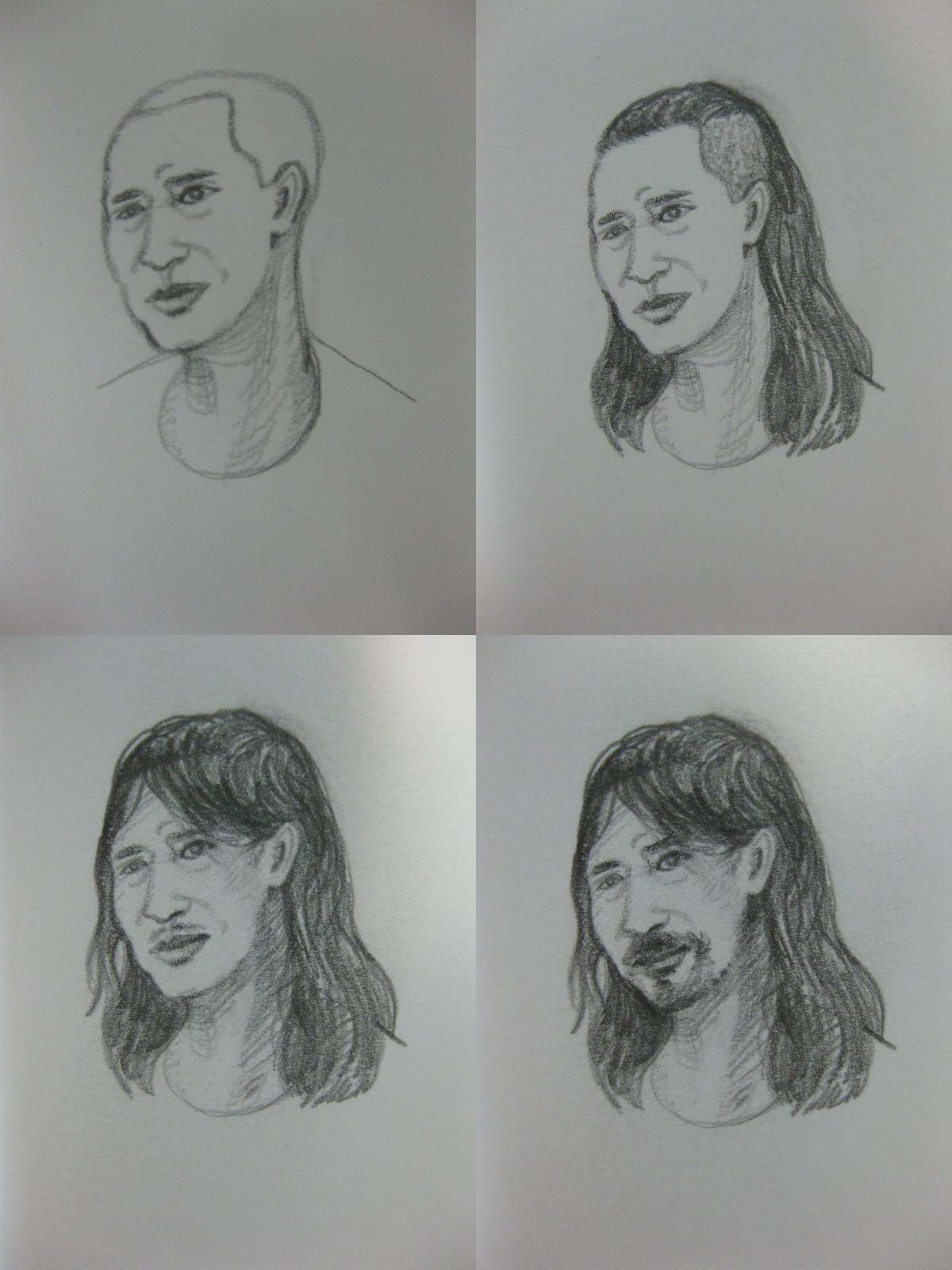This image showcases the progressive stages of a detailed pencil drawing of a man, depicted in a series of four panels arranged in a rectangular format on a blank white sheet. Each panel demonstrates the sequential addition of features and shading, culminating in a richly detailed portrait.

In the top left panel, the initial outlines of the man's face, neck, and shoulders are sketched. Basic facial features are drawn, and the hairline is suggested, but no hair is yet present. The man is facing to the left.

Moving to the top right panel, the drawing shows the addition of preliminary hair, which is long and dark, beginning to fall past the shoulders. Some shading enhances the facial features, providing more depth.

The bottom left panel introduces more detail to the man's hair, adding fullness with bangs and a denser texture around the head. The shading becomes more pronounced, refining the contours of the face and hair further.

Finally, the bottom right panel reveals the completed portrait with significant added detail. The man's hair appears thick and well-defined, reaching his shoulders. New facial details include a scruffy beard and mustache. The shading across the entire drawing is more intricate, creating a realistic and textured look. The man's shirt, which appears black in contrast with the white paper, completes the transformation from a simple outline to a fully realized, black-and-grey pencil drawing.